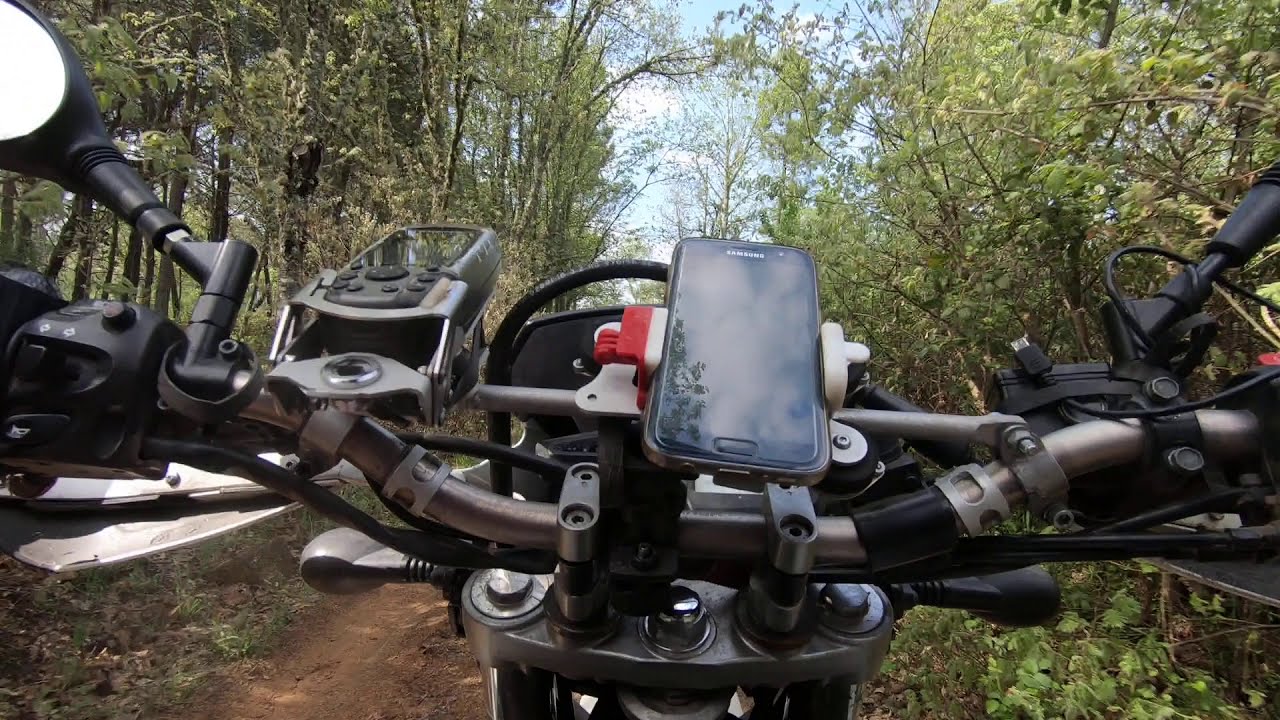The image showcases a first-person perspective from a dirt bike, seemingly captured from a chest-mounted GoPro or action camera. The focus is on the black handlebars of the bike, which feature metallic silver bars and a variety of mounted devices. Central to the handlebars is a phone holder securing a Samsung phone, highlighted by a red and white clip. To the left, there is another mount holding a handheld GPS device. The bike appears to be navigating a dirt trail composed of brown, tan-colored soil, which winds through a dense wooded area. Tall trees brimming with green leaves and branches encircle the path on both sides. Above, the sky is a clear blue adorned with a few high, white clouds, enhancing the idyllic outdoor scene.